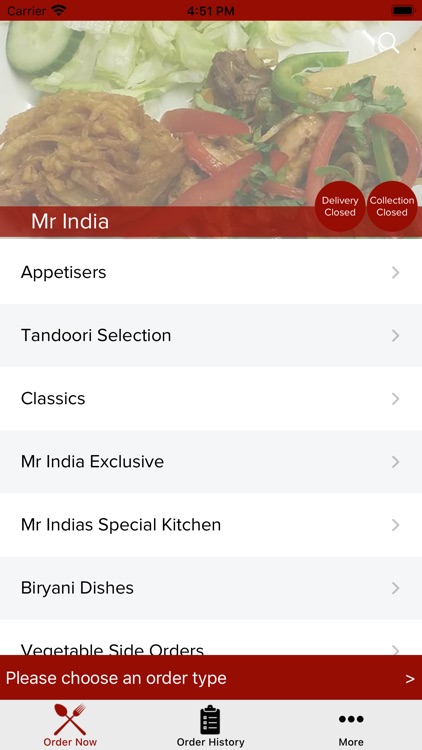A smartphone screenshot captures the interface of an online food ordering platform for a restaurant named "Mr. India". The top of the screen features a red status bar indicating the carrier status as "Carrier" and displays the time as 4:51 p.m., full battery, and Wi-Fi connectivity.

Below the status bar, the app interface contains a vibrant image of a dish comprising various Indian foods, notably adorned with a plentiful array of lettuce, vegetables, peppers, and a mix of chicken and beef.

Prominently situated above the image is the restaurant's name with slightly red highlighting, "Mr. India". Adjacent to the name, on the right side, are two small red circles with white text indicating "Delivery Closed" and "Collection Closed", signifying that the restaurant is currently not accepting orders.

Beneath this information lies the menu selection area, designed with alternating white and light gray backgrounds and black texts categorized as follows: "Appetizers", "Tandoori Selection", "Classics", "Mr. India Exclusive", "Mr. India Special Kitchen", "Biryani Dishes", and "Vegetable Side Orders". Each category has a corresponding gray right-arrow icon next to it, indicating that these are expandable menu options.

Further down the screen, a red bar with white text directs the user to "Please choose an order type" accompanied by a small white arrow pointing to the right.

At the bottom of the interface, three essential navigation options are visible within a menu bar: a red icon with crossed spoon and fork labeled "Order Now", a black text "Order History", and a contrived context menu symbol represented by three dots labeled "More". These navigation options suggest different functionalities such as placing an order, viewing past orders, and accessing additional settings or information.

Overall, the screenshot encapsulates a meticulously designed, user-friendly interface for browsing and ordering from the "Mr. India" restaurant, albeit indicating the current unavailability for both delivery and collection services.